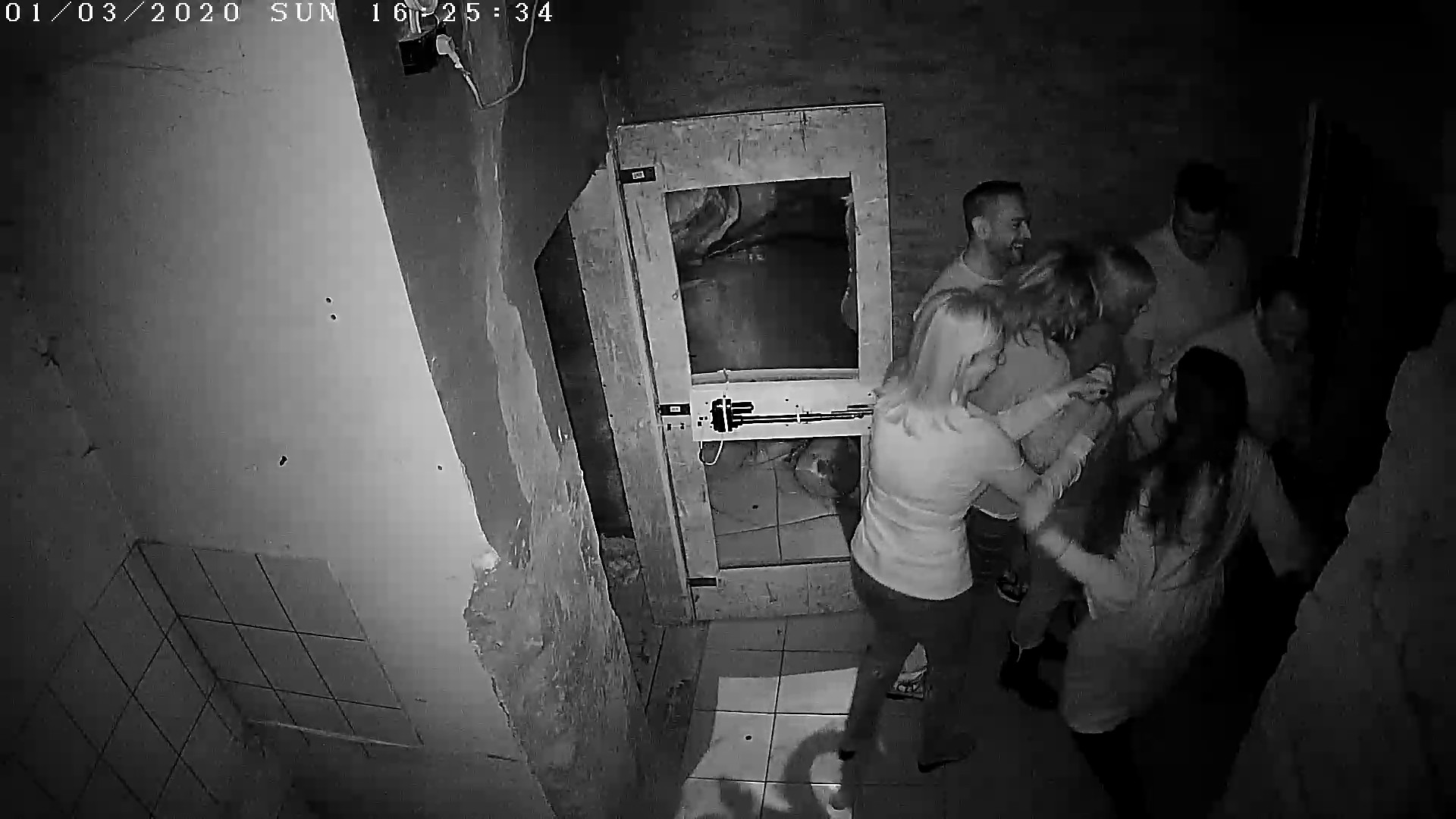The black-and-white image, captured by a security camera, shows a timestamp on the upper left-hand corner reading "01-03-2020, Sunday, 16:25:34." The scene takes place in a dilapidated room featuring a mix of drywall and tile walls showing significant wear, including stains, patches, and deteriorating areas. The floor is made of tiles that extend partway up the walls. A door with mirrors on its interior stands wide open. Seven people, consisting of three men and four women, all wearing white shirts, are gathered in a tight cluster near the door. They appear to be sharing a light-hearted moment, with some laughing and others engaged in playful jostling, as if pushing each other forward. The overall impression is one of a run-down, confined space, possibly a basement, adding a somewhat eerie backdrop to the group's camaraderie.